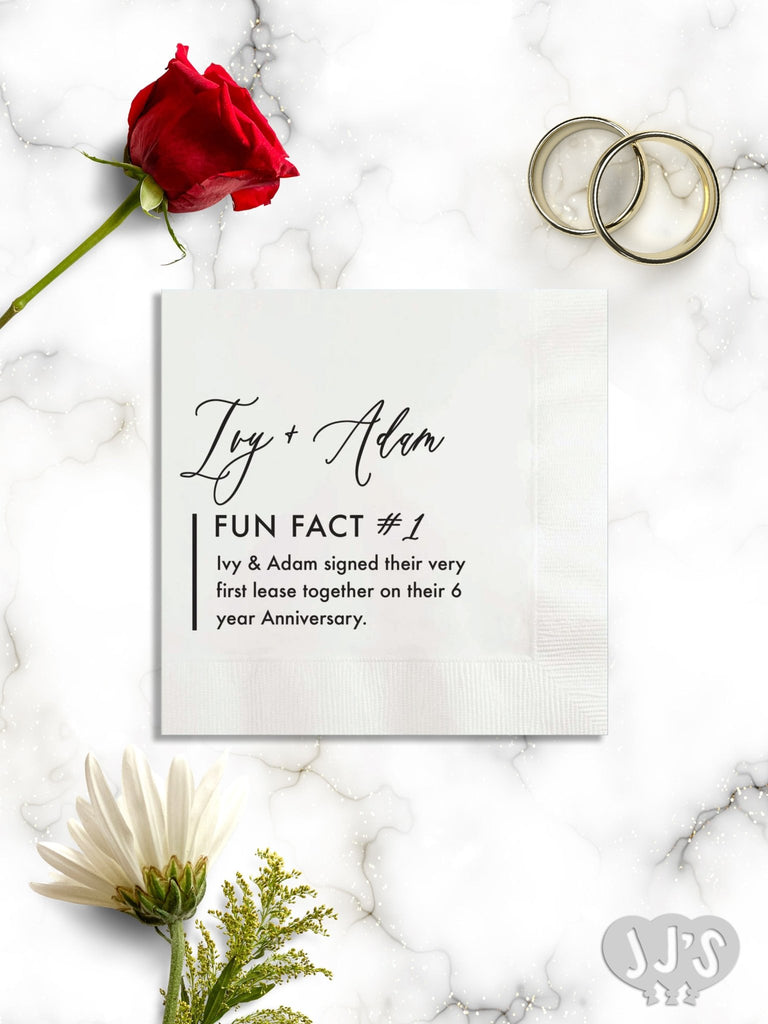The image portrays a meticulously designed graphic centered on an Adam and Eve-themed fun fact. Set against a striking background of white marble marbled with beige veining, the arrangement showcases a variety of elements: 

In the top left corner, a vibrant red rose with a green stem adds a touch of romance. Contrastingly, the top right corner features a pair of intertwined gold rings, symbolic of matrimony. At the center, a white napkin bears the text, "Ivy plus Adam" in elegant black cursive, followed by "Fun Fact number one: Ivy and Adam signed their very first lease together on their sixth anniversary," in plain black text. 

Further enhancing the design, a white flower with a green stem adorns the bottom left corner. The bottom right corner displays a logo, "J.J.S.," stylized to resemble the silhouette of three balloons. The overall palette is a harmonious blend of rose red, green, a range of grays, and metallic hues, which together create a visually captivating and meaningful narrative of a couple celebrating a significant milestone in their relationship.